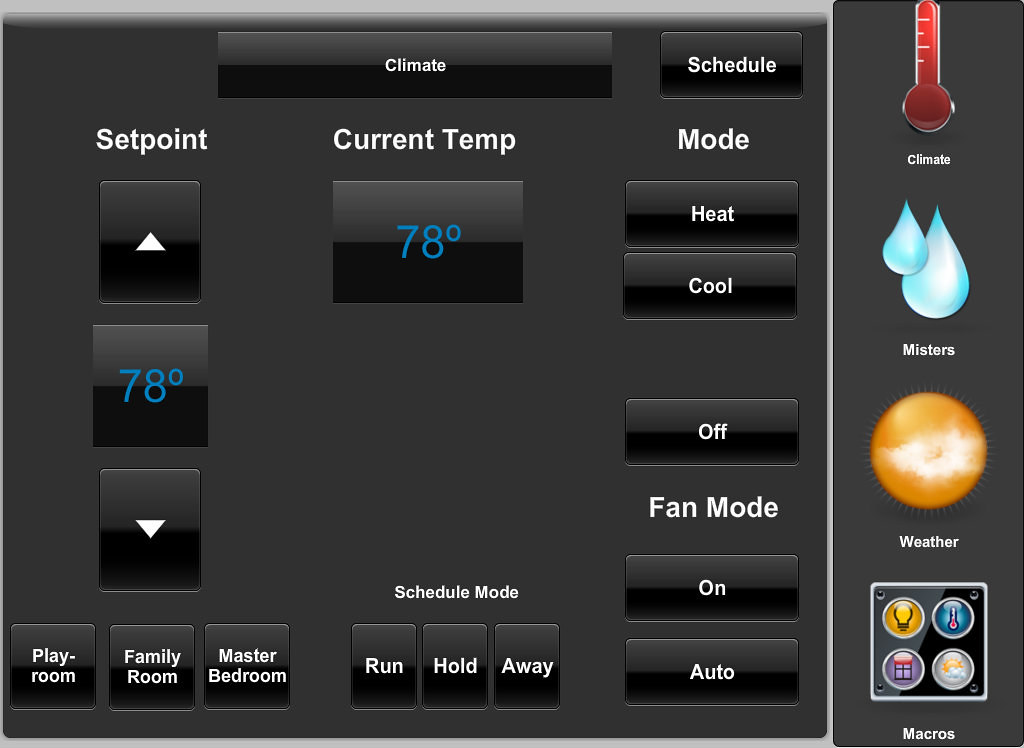In this image, we observe a series of controls and settings displayed on a dark gray background, with a lighter gray section at the top. At the top of the image, there is a rectangular area labeled "Climate" in white text, and to the right of it, a similar rectangle labeled "Schedule." 

Below these, various settings are displayed. On the left side, there are square buttons labeled "Heat," "Cool," "Mode," "Off," "Fan Mode," "On," and "Auto." Directly below these buttons, side by side, are additional square buttons labeled "Schedule Mode," "Run," "Hold," and "Away."

On the left at the bottom, there are buttons labeled "Playroom," "Family Room," and "Master Bedroom," each with a gray top and a black bottom. Above this section is a square containing a white triangle shape, and above that, the text "78 degrees" in blue. Further above, another square with a triangle is marked with "Set Point."

To the right of this, there is a label indicating the "Current Temp" followed by "78 degrees" in blue text. Adjacent to this area, a red thermometer icon is labeled "Climate."

Below this section, there are two water drop icons labeled "Misters," followed by a yellow circle with a white interior labeled "Weather." At the bottom, there are four circles labeled "Macros."